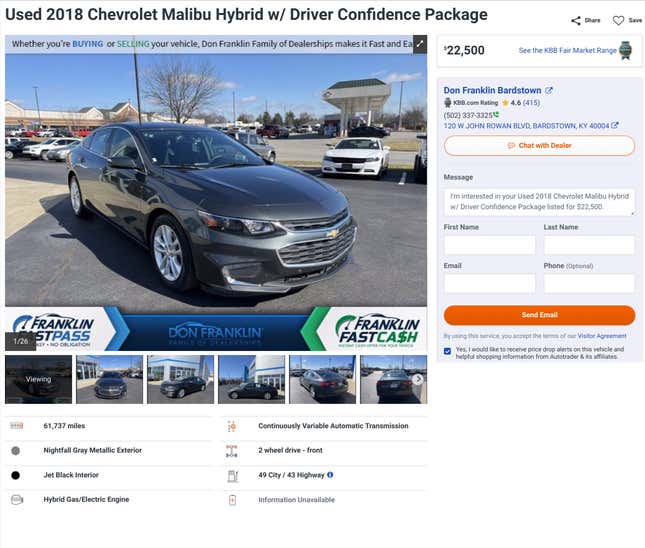**Detailed Caption:**

The image, sourced from the Don Franklin auto dealer's website, features a sleek 2018 Chevrolet Malibu Hybrid sedan in a dark silver or gray finish. Positioned on an outdoor lot presumably next to a grocery store, the car is flanked by other vehicles, including a noticeable white car nearby. The Malibu boasts large wheels and a modern design, appealing to those seeking a stylish yet efficient vehicle.

In the foreground, the Malibu is highlighted from multiple angles, showcasing its front, angled, and side views. Priced attractively at $22,500, the dealership offers a convenient chat option for potential buyers, alongside contact details for Don Franklin of Bardstown. The dealership, located at 120 W. John Rowan Boulevard in Bardstown, Kentucky, boasts a commendable 4.6-star rating. Interested customers can reach out via phone at 502-337-3325 or through a provided message form requiring basic information like name, email, and phone number.

Don Franklin's website also promotes their Franklin Fast Cash Program and Franklin Fast Pass, aimed at expediting the car buying or selling process. The Malibu on display further includes the Driver Confidence Package, increasing its appeal to safety-conscious buyers. Additionally, the site offers a range of 26 photos of the vehicle and provides the Kelley Blue Book (KBB) market range to ensure transparent pricing. Options to save or share the listing enhance user convenience. Overall, this detailed presentation underscores the dealership’s commitment to making vehicle transactions swift and hassle-free for their customers.